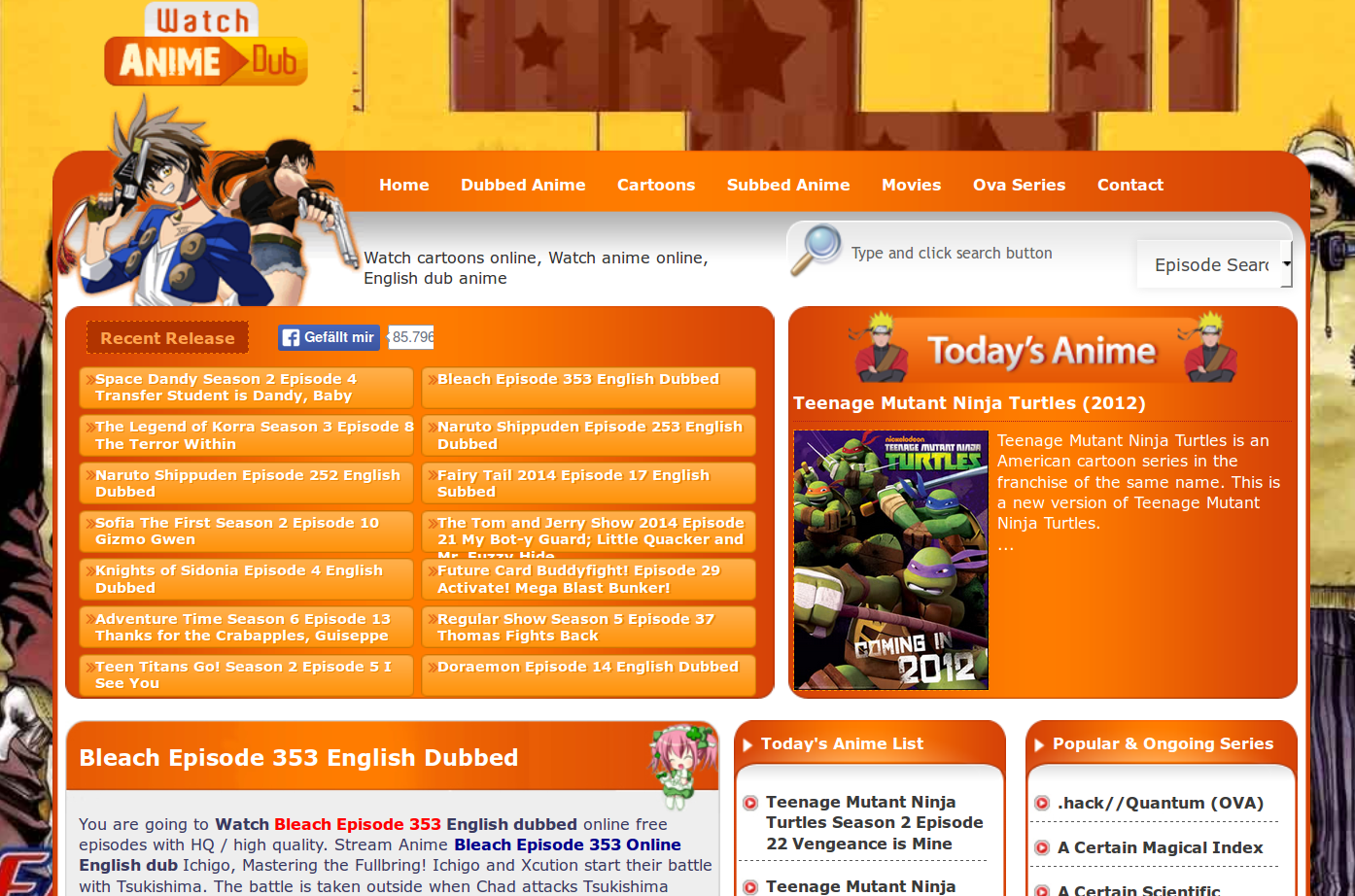The image showcases a vibrant website dedicated to promoting dubbed anime. The website features a colorful, cartoon-inspired design with a playful palette of oranges, greens, purples, and whites. 

On both the left and right sides of the page, there are illustrated characters that enhance the whimsical appearance. In the center, a prominent pop-up announces "Today's Anime: Teenage Mutant Ninja Turtles (2012)". The pop-up displays two women at the top; one with spiky gray hair, a crop jacket, and holding a gun near her forehead, while the other sports jean shorts, a tank top, and a ponytail, holding a large gun.

At the top of the page, a bright orange navigation bar lists options such as Home, Dubbed Anime, Cartoons, Subbed Anime, Movies, OVA, Series, and Contact. Below this section, the main body highlights recent releases in vibrant orange text.

A large box prominently displays "Today's Anime" with a Teenage Mutant Ninja Turtles feature. Beneath this, there's information about "Bleach Episode 353, English Dubbed," accompanied by a brief description. Adjacent to these sections, there are categories for "Today's Anime List" and "Popular and Ongoing Series."

The website also includes a white search box where users can type queries and click the search button. This detailed and colorful layout makes it easy for users to explore a variety of anime options in a visually engaging way.